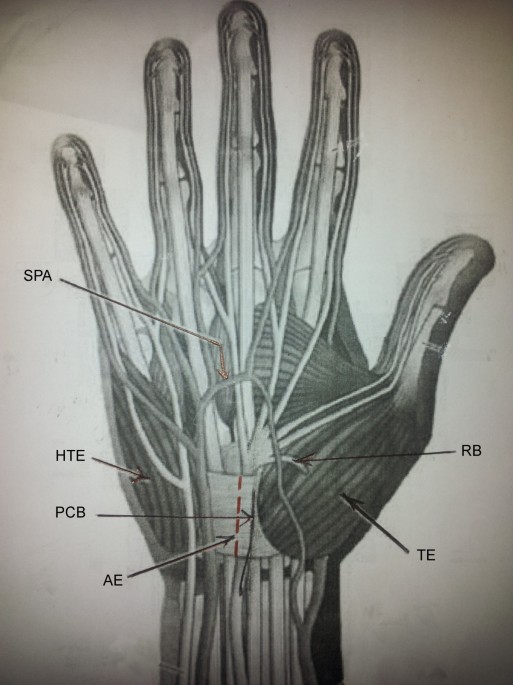This detailed black-and-white diagram depicts the anatomy of a left human hand with the skin removed to reveal the underlying muscles, tendons, and bones. The palm is prominently displayed, highlighting the intricate network of muscle fibers and tendons that extend into the fingers. The background is a creamy white with subtle shadowing, emphasizing the contrast. Labels using two or three-letter codes, such as TE, HTE, PCB, AE, SPA, and RB, are strategically placed pointing to various anatomical structures from top left to bottom right. The image is reminiscent of a highly detailed pencil drawing, giving it a digital yet traditional illustrative feel. The hand extends with all five fingers spread, and the diagram stops just above the wrist, making it a comprehensive visual guide likely suitable for medical educational purposes.